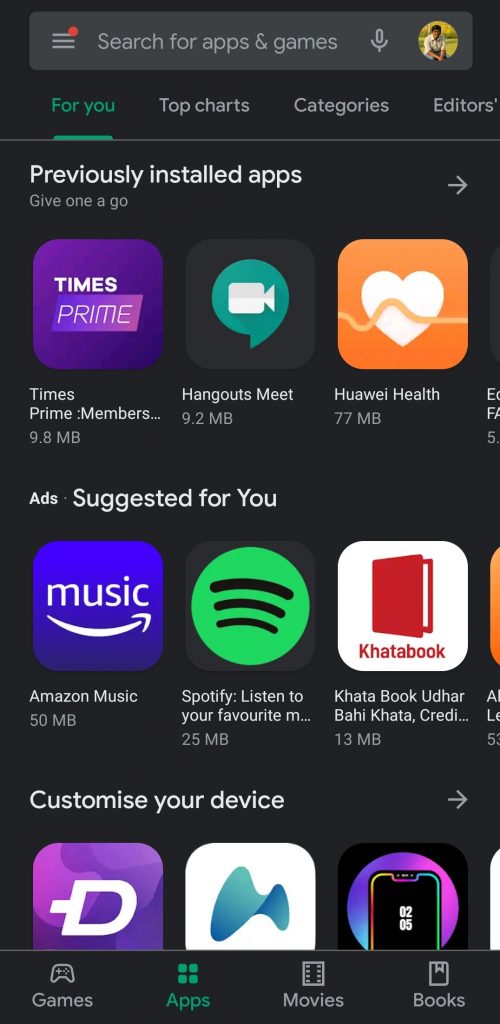This is a detailed screenshot of a smartphone displaying the "Search for apps and games" page. At the top left, there's a hamburger menu icon. In the top right corner, the user's profile photo is displayed inside a circular icon. Between these, a search bar reads "Search for apps and games," with a microphone icon immediately to its right.

Below the search bar, there are several tabs: "For You," which is the currently selected tab, "Top charts," "Categories," and part of a cut-off tab presumably labeled "Editor's pick." 

Directly beneath the tabs, the section titled "Previously installed apps - Give one a go" appears, featuring a right-facing arrow on the right side. In this section, three apps are listed:
1. Times Prime - 9.8 MB
2. Hangouts Meet - 9.2 MB
3. Hoy Health - 77 MB

Following this, there's a section labeled "Ads suggested for you," including the following apps, each with its associated details:
1. Amazon Music - 50 MB
2. Spotify: Listen to your favorite music - 25 MB
3. Kata Book: Udhar bahi, Kata, credit... - 13 MB

Further down, there's another section titled "Customize your device" with a right-facing arrow. This is followed by three more icons, whose names are unreadable as they are partially cut off by the screen's bottom border.

At the bottom of the screen, a navigation bar includes icons for "Games," "Apps" (which is highlighted in green, indicating the current page), "Movies," and "Books."